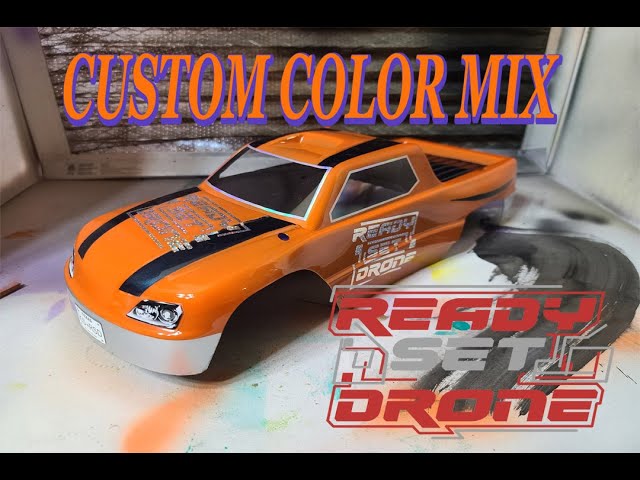The image features an advertisement framed by a black border at the top and bottom. Below the top black border, large orange capital letters with a slight purple edging spell "CUSTOM COLOR MIX." Underneath this text, the focal point is a picture of a light gray, dirty floor vent that extends upwards off the image, just touching the black border. Beneath the vent, a light-colored floor provides contrast.

Dominating the middle section of the image is the orange body of a car, closely resembling an El Camino truck. This vehicle appears to be a model or perhaps a drone cover—lacking wheels and inner workings, emphasizing its shell-like appearance. The car sports two prominent black stripes running along its hood and roof. On the visible driver's side door, the words "READY SET DRONE" are inscribed in white lettering.

In the bottom right-hand corner, bold red letters spell "READY," followed by "SET" in gray, and "DRONE" in red once more, forming the phrase "READY SET DRONE." This text adopts a robotic font and is accompanied by gray streaks that arc upward and then curve back, culminating near the left rear wheel well of the car body. The overall composition underscores a modern, dynamic aesthetic fitting for a tech-focused advertisement.